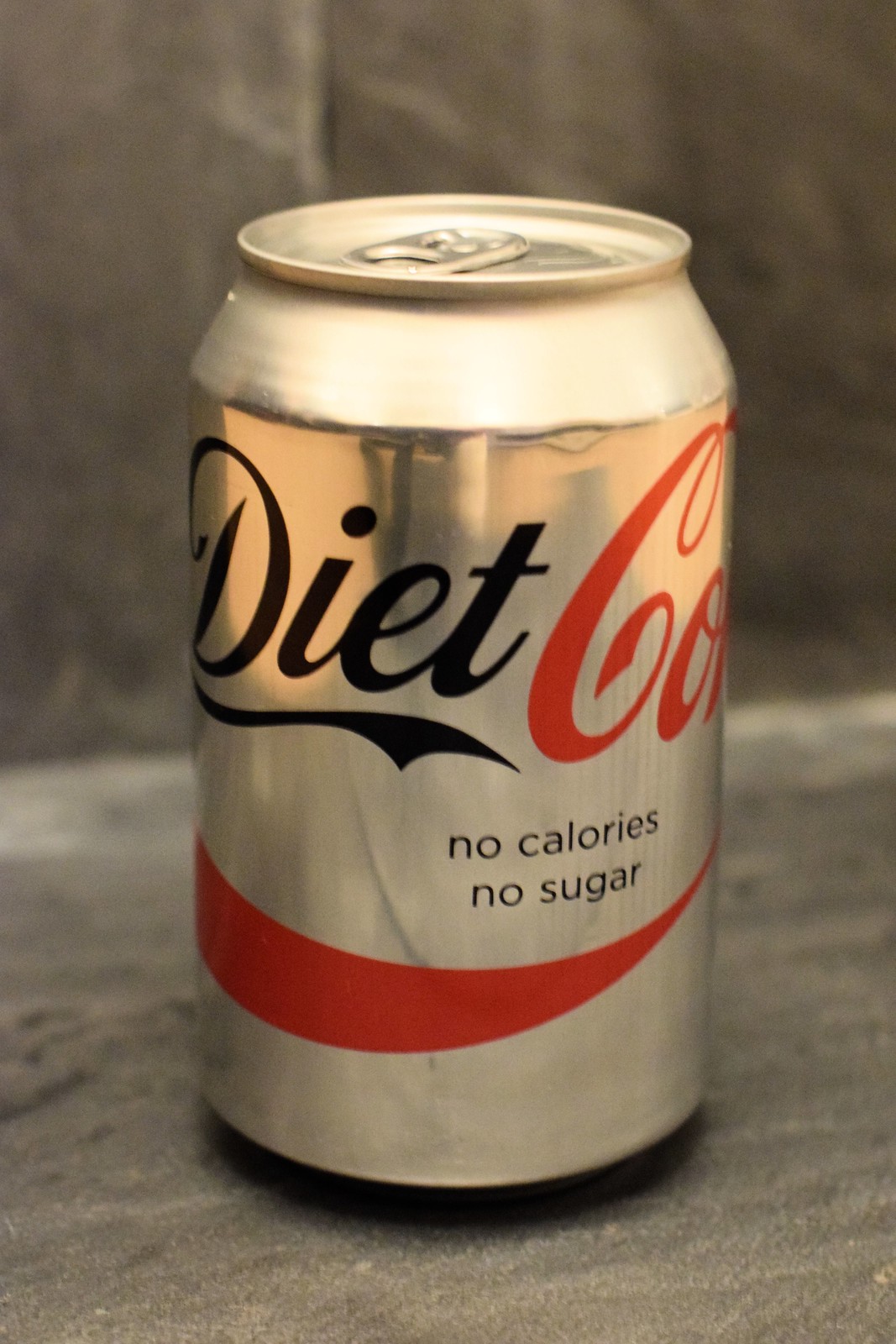The image features an unopened Diet Coke can prominently positioned low to the ground, suggesting it is resting on a surface that appears to be outdoors. The can maintains its recognizable design, with the word "Diet" printed in black and "Coke" in bold red lettering. The can is silver, reflecting its classic sleek style, and is marked with "No calories, no sugar" in clear text. At the bottom of the can, a red emblem reminiscent of the iconic Coca-Cola logo is visible, characterized by a simple red line. The background consists of large, rugged stones or rocks, enhancing the natural outdoor setting implied by the lighting and texture of the surroundings. No people or extraneous objects are present, keeping the focus solely on the Diet Coke can, which embodies the quintessential branding and visual identity associated with Coca-Cola products.